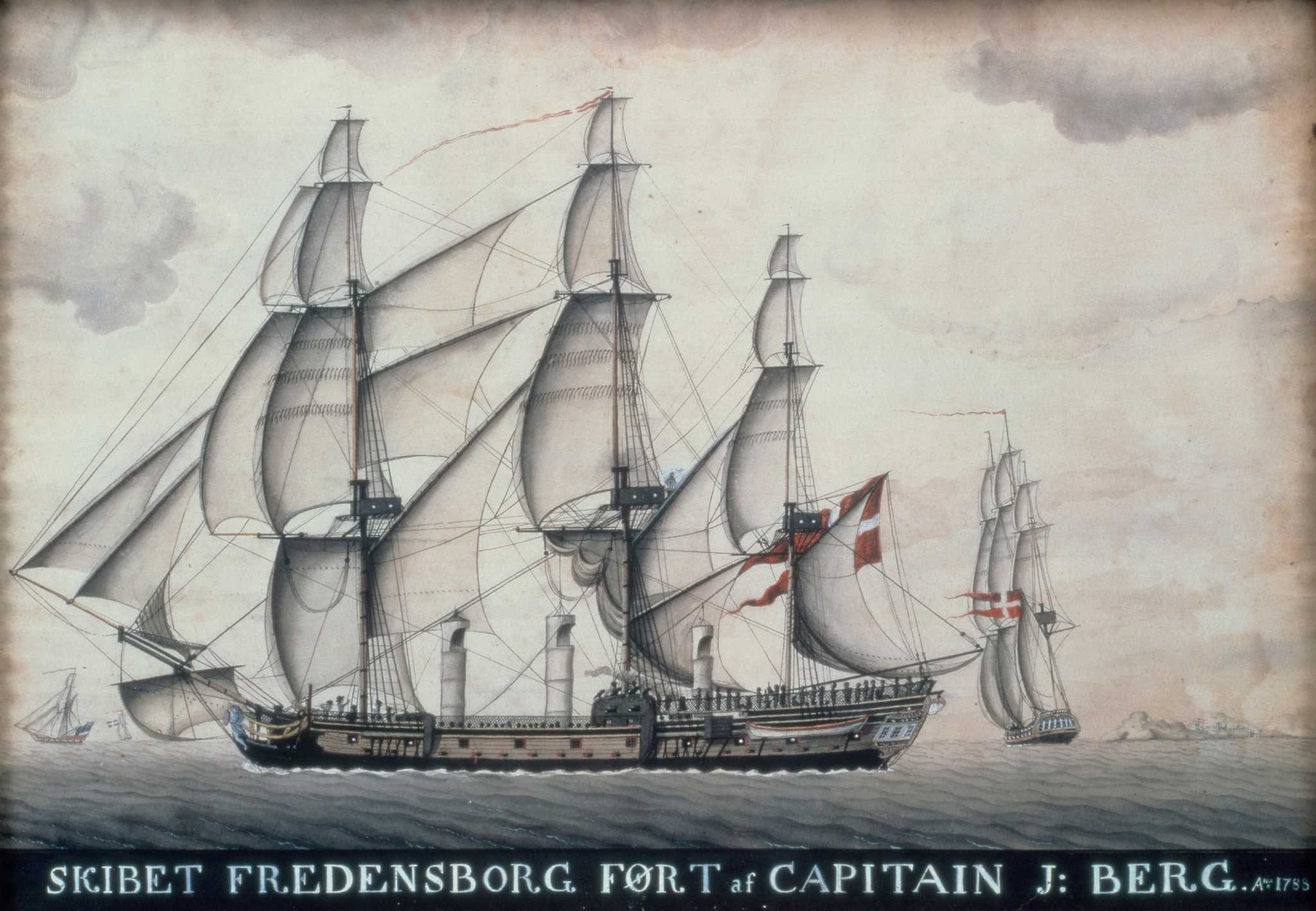This square, color illustration captures an 18th-century tall ship named "Skibet Fredensborg Fort AF Captain J. Berg," prominently inscribed at the bottom. The ship, dated Anno Domini 1755, showcases triple masts with numerous sails, and an additional sail towards the rear. Onboard, there are three peculiar white towers. The vessel is an open wooden boat, and at its stern, partially concealed by a sail, flies a Danish flag. The background is a nuanced beigey gray with hints of pink, featuring a grayish sea. To the right of the central ship is another similar tall ship, adorned with a white and red flag and a maroon and white flag atop. Additionally, a smaller vessel is visible on the left. The upper sky segment appears mostly white with scattered gray clouds towards the top. The entire scene evokes a historical maritime setting, complete with detailed rigging and atmospheric color tones.